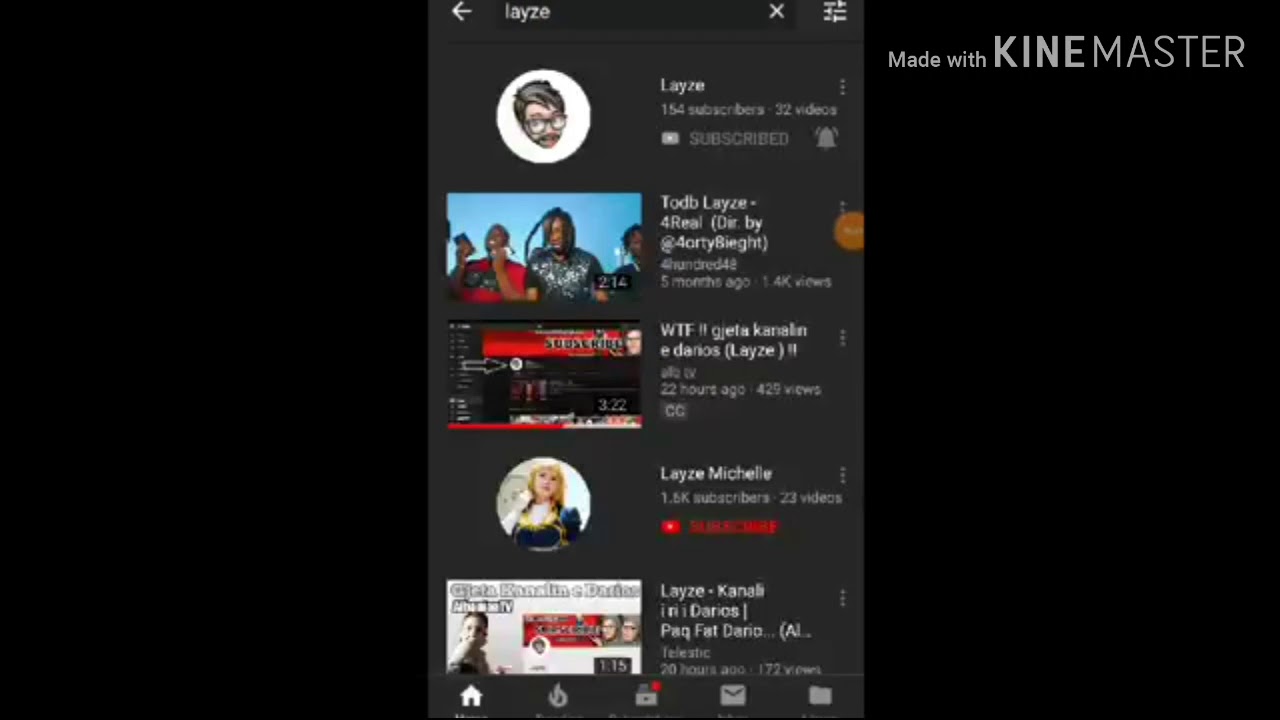A rectangular, black background with the "KineMaster" logo in white text located at the upper right corner. Centrally placed on the image is a strip that resembles a cell phone screen displaying the following details:

- **Upper Left Corner**: The word "Lazy" written as "L-A-Y-Z-E".
- **Left Side**: An arrow pointing to the left.
- **Upper Right Corner**: A box that resembles a 'close' button or an 'X'.
- **Below the Box**: "Lazy", "154 subscribers", "32 videos", and a "Subscribe" button.
- **Middle Section**: "Toby Lazy 4Wheel", and "Directed by ARTIE SIGHT".

Beneath these details, it reads "five months ago.” Below this, another video detail is visible: “WTF! Greta Kansln".